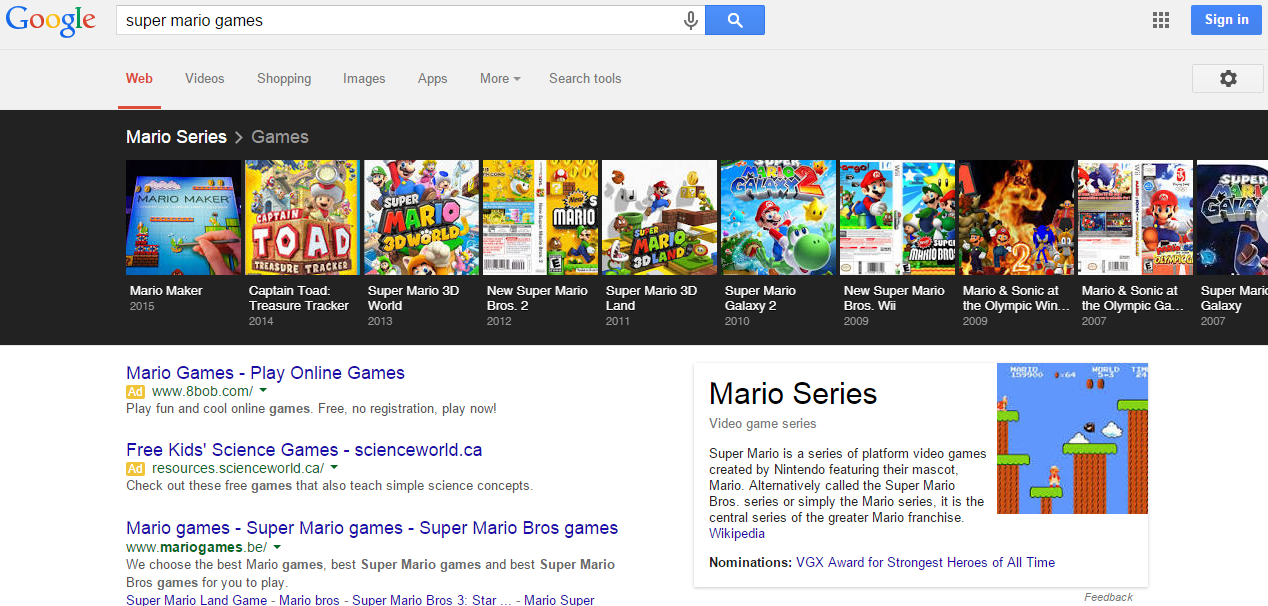The image is a screenshot of a Google search results page for the query "Super Mario Games." The main portion of the image displays a series of web results, each with corresponding game cover images and titles beneath them. The featured games include:

1. "Super Mario Maker" (2015)
2. "Captain Toad: Treasure Tracker"
3. "Super Mario 3D World"
4. "New Super Mario Bros. 2"
5. "Super Mario 3D Land"
6. "Super Mario Galaxy 2"
7. "New Super Mario Bros. Wii"
8. "Mario and Sonic at the Olympic Games" (partially cutoff titles: "Mario and Sonic at the Olympic Win..." and "Mario and Sonic at the Olympic GA...")
9. "Super Mario Galaxy" (partially cut off title)

Beneath these game covers are additional search results, including:

- An advertisement titled "Mario Games, Play Online Games," with a website link provided.
- Another ad for "Free Kids Science Games," promoting educational games that teach simple science concepts with a linked web address.
- A non-sponsored search result titled "Mario Games, Super Mario Games, Super Mario Brothers Games," highlighting selected Mario games with a web address.

On the right side of the page, there is a rectangular section containing text that reads "Mario Series, Video Game Series," alongside a screenshot from one of the Mario games.